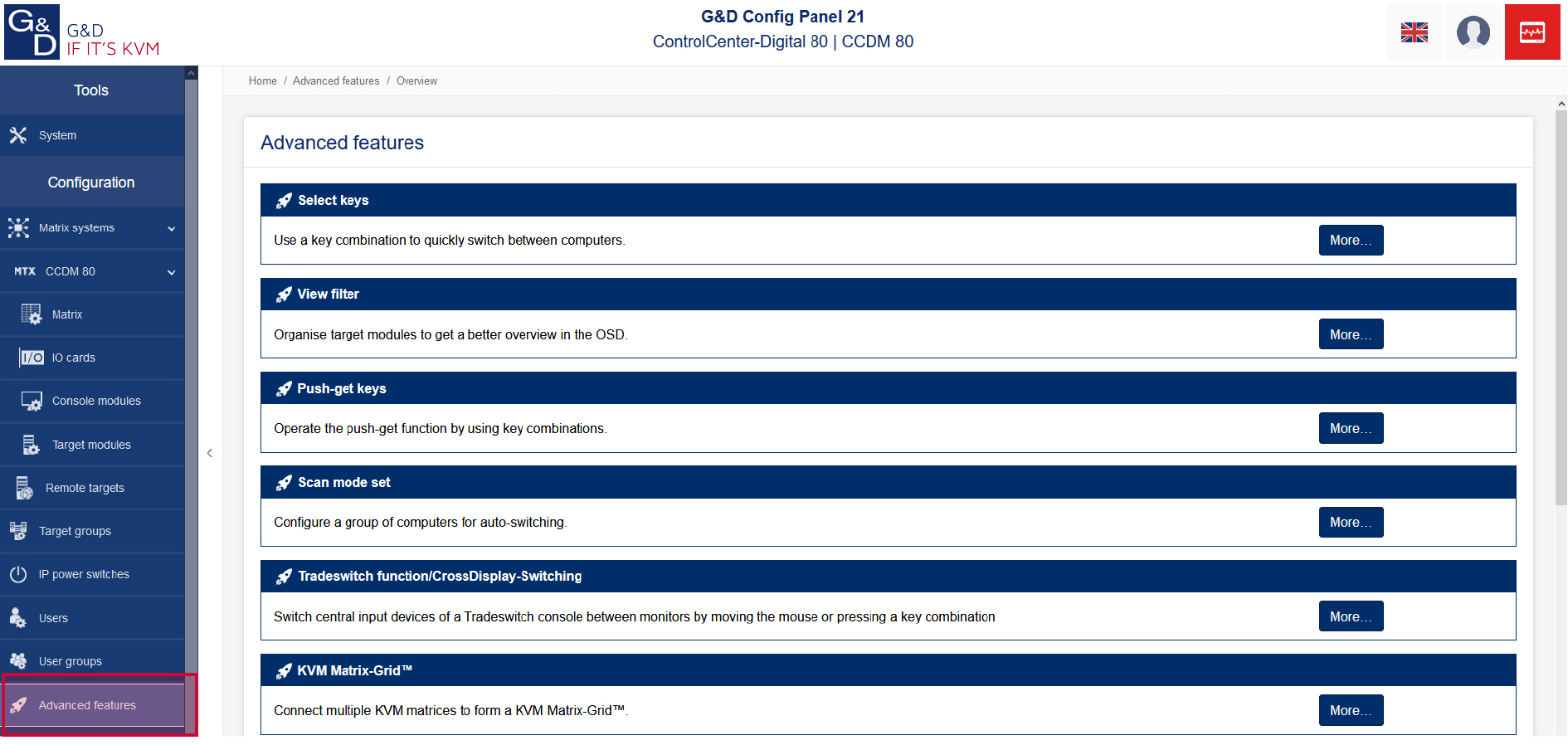Here is the detailed and cleaned-up caption for the image:

---

The image features a detailed interface for a website dedicated to "G&D." It presents a blue square background with bold white text at the top displaying "G&D," alongside the KVM symbol. Below this header, a structured column lists various options, each enclosed in a blue box with white text. The options include: 

- Tools
- System 
- Configuration
- Matrix Systems 
- CCOM 60 Matrix 
- ID Cards
- Console Modules 
- Target Modules 
- Remote Targets 
- Target Groups 
- IF Power Switches / IP Power Switches 
- User 
- User Groups

The final entry, "Advanced Features," stands out, highlighted in a red box. To the right of this column, a wider section outlines a series of rows alternating between white and navy blue backgrounds. At the top of this section, it reads "G&D, Config Panel 21, Control Center - Digital 80, CCDM 80, Home, Advanced Features Overview."

Within this field, a specific area on a white background with blue text lists several advanced features:

- A navy blue bar titled, "Select Keys," accompanied by a rocket ship icon
- An instruction stating, "Use a key combination to quickly switch between computers"
- A view filter shown to, "Organize target modules to get a better overview in the OSD"
- Push Key and Push Get Keys for operating the push-get function using key combinations
- "Scan Mode Set," allowing configuration of computer groups for auto-switching
- "Trade Switch Function," with cross-display switching abilities for shifting central input devices across a trade switch console by moving the mouse or using a key combination
- "KVM Matrix Grid," which facilitates the connection of multiple KVM matrices to form a KVM matrix grid

In the upper right-hand corner of the image, three icons are displayed: a British flag, a person, and a red square box.